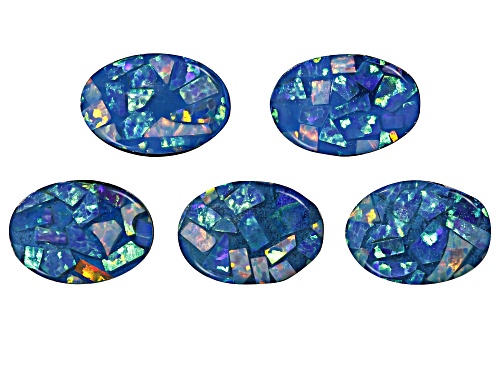The image depicts five handmade, circular mosaic-like pieces set against a white background. These vibrant circles, arranged with two at the top and three at the bottom, feature intricate and colorful designs made from broken pieces of glass or stone. Primarily dominated by shades of blue, the designs also incorporate pops of pink, purple, green, yellow, orange, and white. The small, irregularly shaped tiles are artfully glued to dark blue backgrounds within each circle, creating an eye-catching and reflective display. The intricate arrangement and variety of colors suggest that these pieces are intended for decorative purposes.